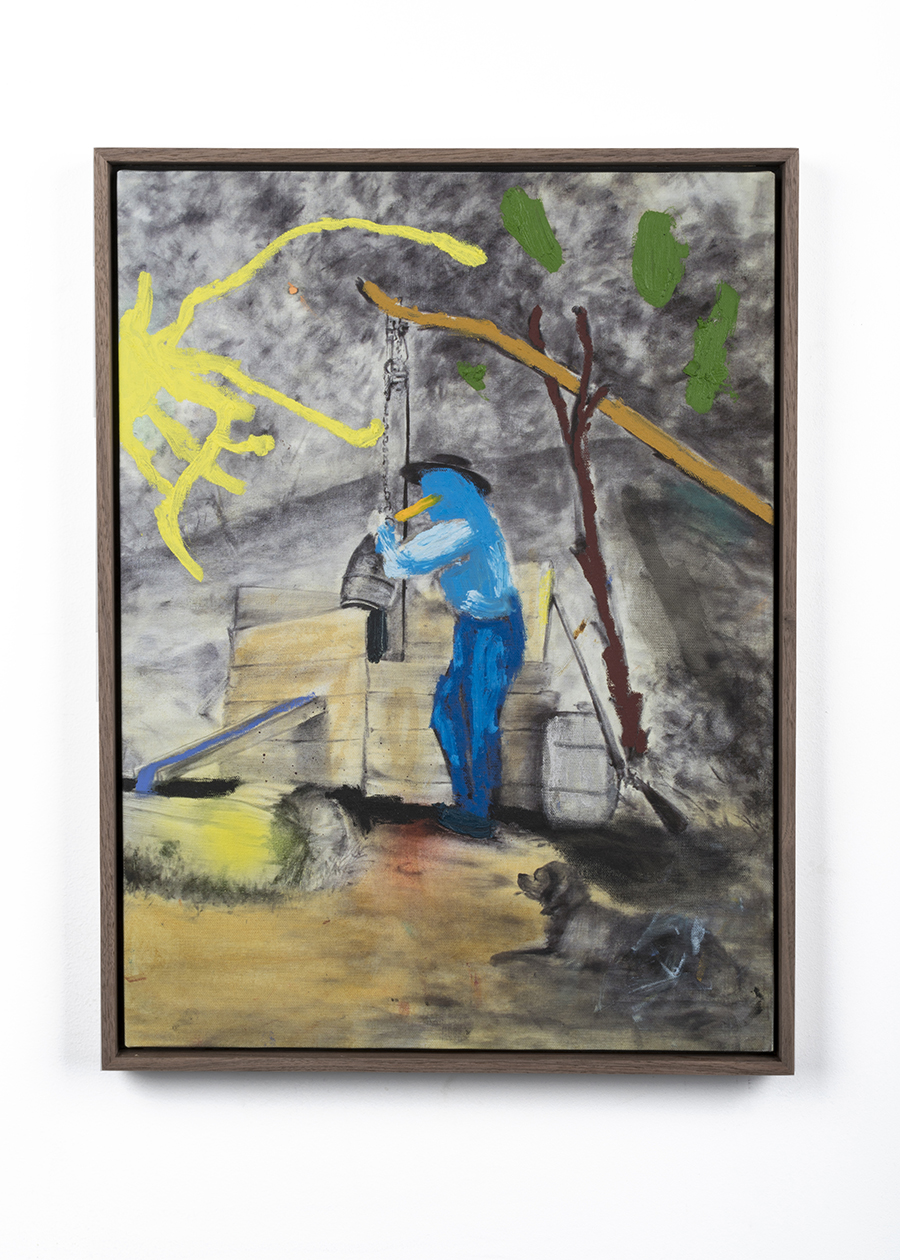This is a detailed painting that balances between realism and abstraction, showcasing a fisherman dressed in blue, wearing blue jeans and a black-rimmed cowboy hat. The fisherman stands by a small wooden boat in the water, engaged in pulling water out of a well with a makeshift crane constructed from a stick and a tree. A brown dog sits in the grass nearby, adding a touch of realism. Bright yellow lines and green splotches representing trees contrast against the dark, textured background of heathered black and white. The painting features a mix of bold colors and impressionist style, giving it an overall textural and somewhat abstract feel.